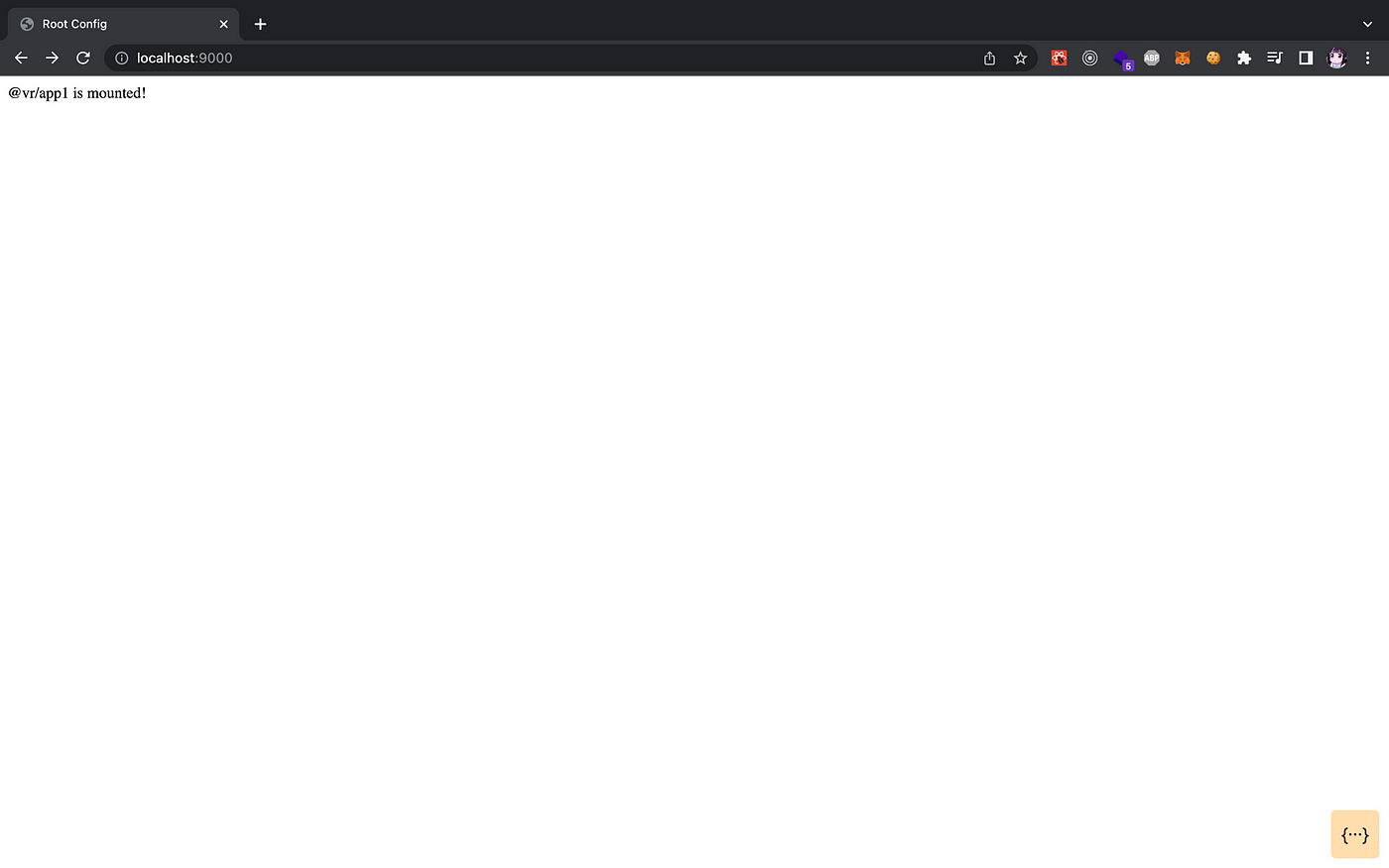Screenshot of an open Google Chrome browser window. At the top, a black bar displays the tab name "rootconfig" in white font, with the URL indicating "localhost:9000." To the right of the tab name, there's a small icon for bookmarking, followed by several other bookmark icons. Below the address bar, the main display area is almost entirely white, except for a small line of black text in the upper left corner that reads "vr/appa1 is mounted!” In the lower right corner of the screen, there is a small, light orange square containing two black brackets with three apostrophes in between them.